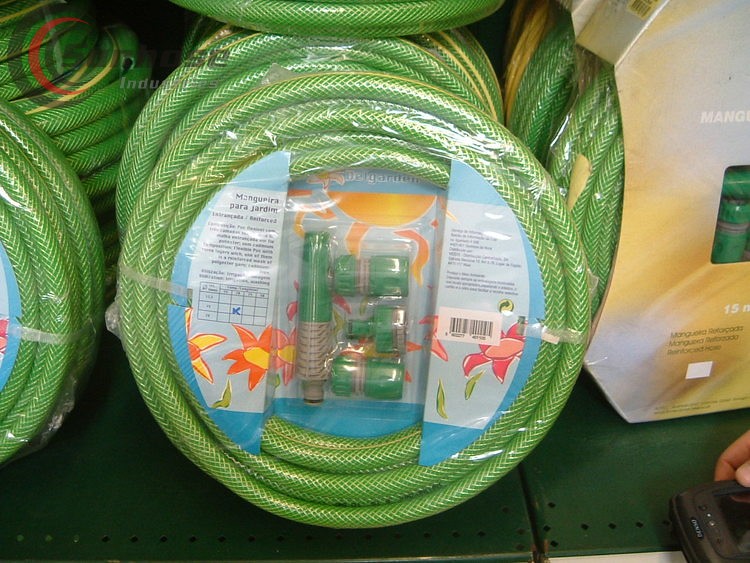In this image taken inside a store, most likely a hardware store, a selection of garden hoses is displayed on shelves. The hoses are light green in color, coiled up, and wrapped in plastic. Each pack features a light blue label in the middle of the coiled hose. Inside the plastic wrap, several types of nozzles and attachments can be seen. There are four nozzles in total: one long cylindrical attachment likely for the end of the hose, and three shorter ones that appear to be faucet adapters or extensions. These short nozzles could be used to fit various faucet sizes. The hoses are stacked and leaning against each other, with additional bundles visible in the background, arranged horizontally. In the top left corner of the image, there is a watermark featuring a red and black circle with partially legible text reading "S-E-N" and "S-E." A hand holding a black object is also slightly visible in the picture, adding a hint of human presence.